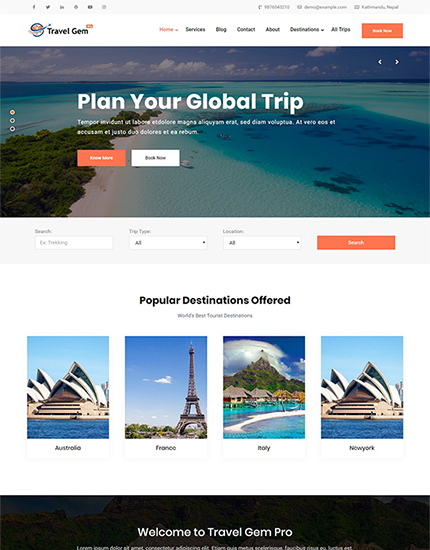This is a detailed screenshot of a website called Travel Gym. At the top left, various social media icons are prominently displayed. Just below these icons, the site's logo is visible, displaying "Travel Gym" in black text. Adjacent to the logo, there is a navigation menu with options labeled Home, Services, Blog, Contact, About, Destinations, and All Trips, followed by an orange button with white text.

Beneath the menu, the page features a captivating picture of a beach, showcasing mostly the ocean, a sliver of sandy shore, and a light grassy area under a partly cloudy sky. Above this beach photo, bold white text commands attention with "Plan Your Global Trip." Directly below this headline, smaller white text provides additional details, flanked by an orange button and a white button for user interaction.

Further down the page, users can input their trip preferences through a search box with fields for trip type and location, accompanied by a search button. Underneath, in black text, the section titled "Popular Destinations Offered" introduces four enticing destination photos: Australia, France, Italy, and New York.

At the bottom of the page, a black bar runs across the width, containing welcoming white text that reads, "Welcome to Travel Gym Pro."